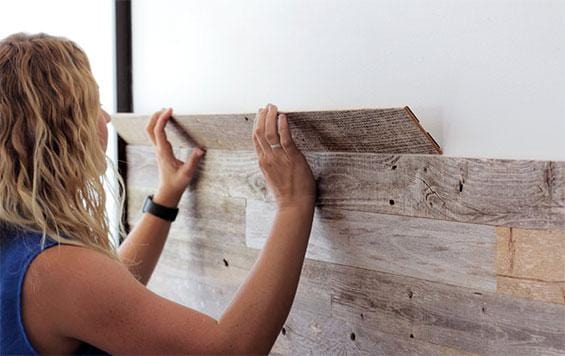In the photograph, a blonde woman with wavy hair is seen in the bottom left corner, facing a white wall as she meticulously installs wood paneling. The thin, aged-looking wood pieces she is setting onto the wall vary in shades of gray, white, and tan, giving the wall a rustic, character-rich appearance. She is carefully positioning a board on top of previously aligned panels, ensuring a snug fit. The woman is dressed in a blue, sleeveless shirt—or possibly a denim tank top—and wears a black wristwatch on her left hand and a wedding ring on her right ring finger. Visible from the side, her concentration is clear, though her eyes are not visible. Behind the paneling, a dark strip of wood or metal serves as a rail, guiding her installation efforts.